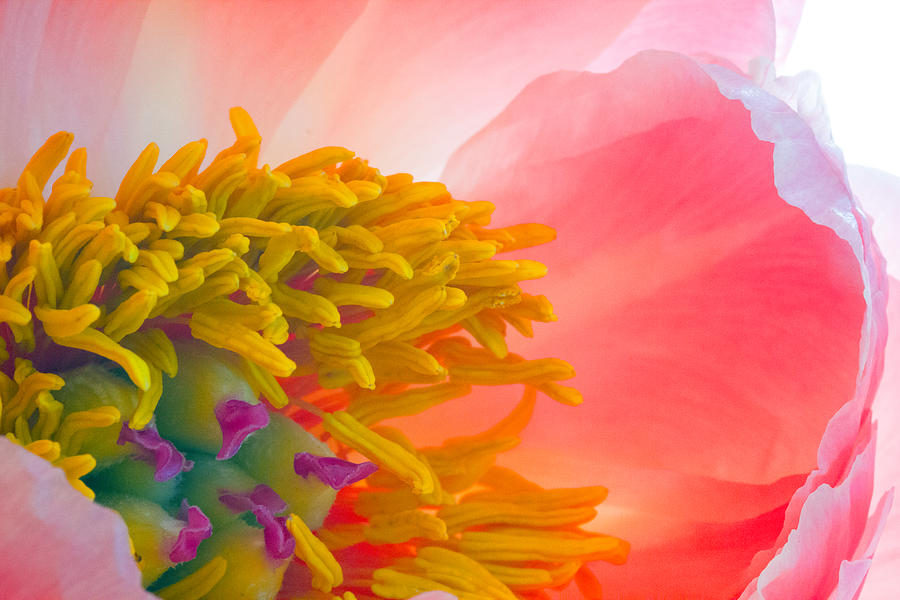The image is a close-up, artsy shot capturing the vibrant and detailed center of a flower, resembling a painting. The dominant focus is on the pollen-coated yellow hairy structures, which encircle small green nubs crowned with squiggly fuchsia tips. The surrounding petals, bathed in sunlight, display a delicate gradient of light pink and peach hues, creating a harmonious blend with waves of mixed pink, white, and peach in the background. The flower’s off-centered positioning adds a dynamic compositional element, drawing attention to the vividly detailed interior that resembles an anemone. The image employs a bright pastel palette of pinks, peaches, lavenders, yellows, purples, and greens, giving it a vibrant, almost luminous appearance, suggesting it could be rendered in either watercolors or possibly oils.